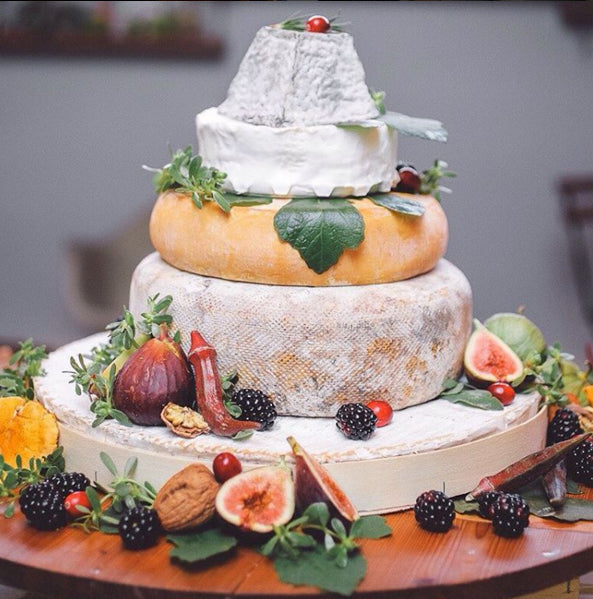This color photograph depicts a meticulously arranged tower of cheese wheels, designed for an elegant cheese and fruit board presentation. The foundation of the tower is a wide cheese wheel with a dusty white rind, mottled with orange areas and featuring a heavily textured crust. Atop this is a slightly smaller wheel of orange cheese, followed by a round wheel of cheddar-like cheese with a similar white rind. A creamy white cheese, resembling brie without the powdery exterior, is next, and the pinnacle of the tower is capped with a conular or bun-shaped cheese dusted in white. Adorning the cheese tower are various decorative elements, including leaves, sprigs of parsley or mint, and an assortment of fruits such as blackberries, figs (both whole and halved), and red berries, adding vivid splashes of color. This entire arrangement sits on a wooden tray in front of a gray background, creating a visually captivating centerpiece for any entertaining occasion.